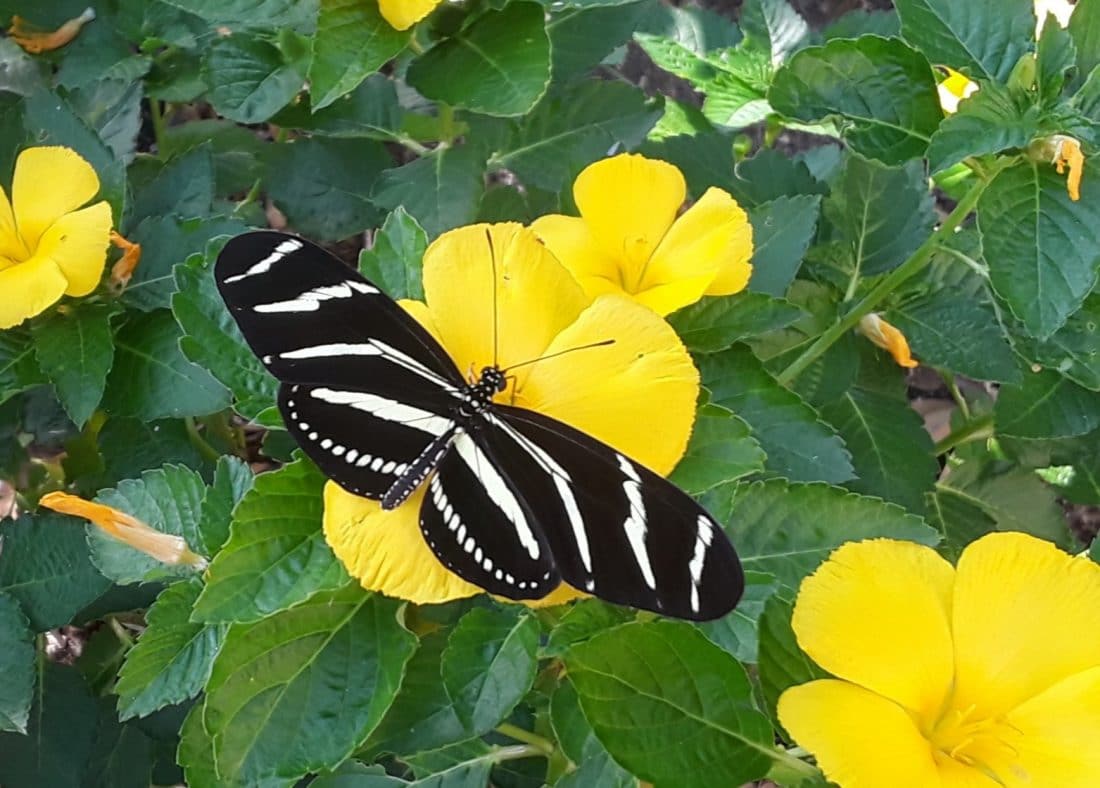This is an overhead photograph of a striking black and white zebra butterfly perched on a vivid yellow nasturtium flower amidst lush green foliage. The butterfly, centrally positioned, showcases its beautiful black wings adorned with distinctive white stripes and dots. It has its antennae clearly visible, adding to the intricate details of its body. Surrounding the butterfly are three other vibrant yellow nasturtium flowers — one to the top left, one to the bottom right, and one just above the center flower. The plant is also dotted with several green leaves and flower buds. The only colors in the photograph are the stark black and white of the butterfly, the bright yellow of the flowers, and the rich green of the leaves, creating a visually captivating contrast.